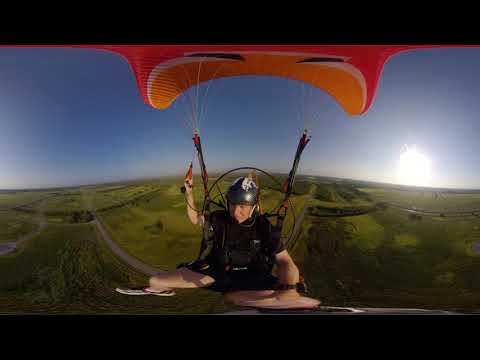The low-resolution, panoramic photograph features a person, identifiable as a man with a Caucasian complexion and wearing a black short-sleeved shirt, black shorts, and a black helmet, who is paragliding. He is positioned near the center, slightly towards the bottom of the image, and is harnessed to a parachute. The harness includes thick black ropes that separate into smaller white ropes connecting to an obscured parachute at the top of the image. The parachute's vibrant colors—comprising orange, reddish-pink, white stripes, and some dark blue elements—add a striking contrast to the scene.

The background reveals a landscape of green fields with varying shades of green, bisected by a few visible roads. The view is slightly warped near the bottom, causing some distortion, particularly noticeable in the man's bare legs. Above this rural expanse stretches a clear blue sky, transitioning from a darker blue near the center to a lighter hue near the horizon. A bright sun, either rising or setting, is visible near the right side, adding a dramatic lighting effect to the image. The top and bottom of the photograph are bordered by thick black rectangles, framing this breathtaking yet distorted aerial view.